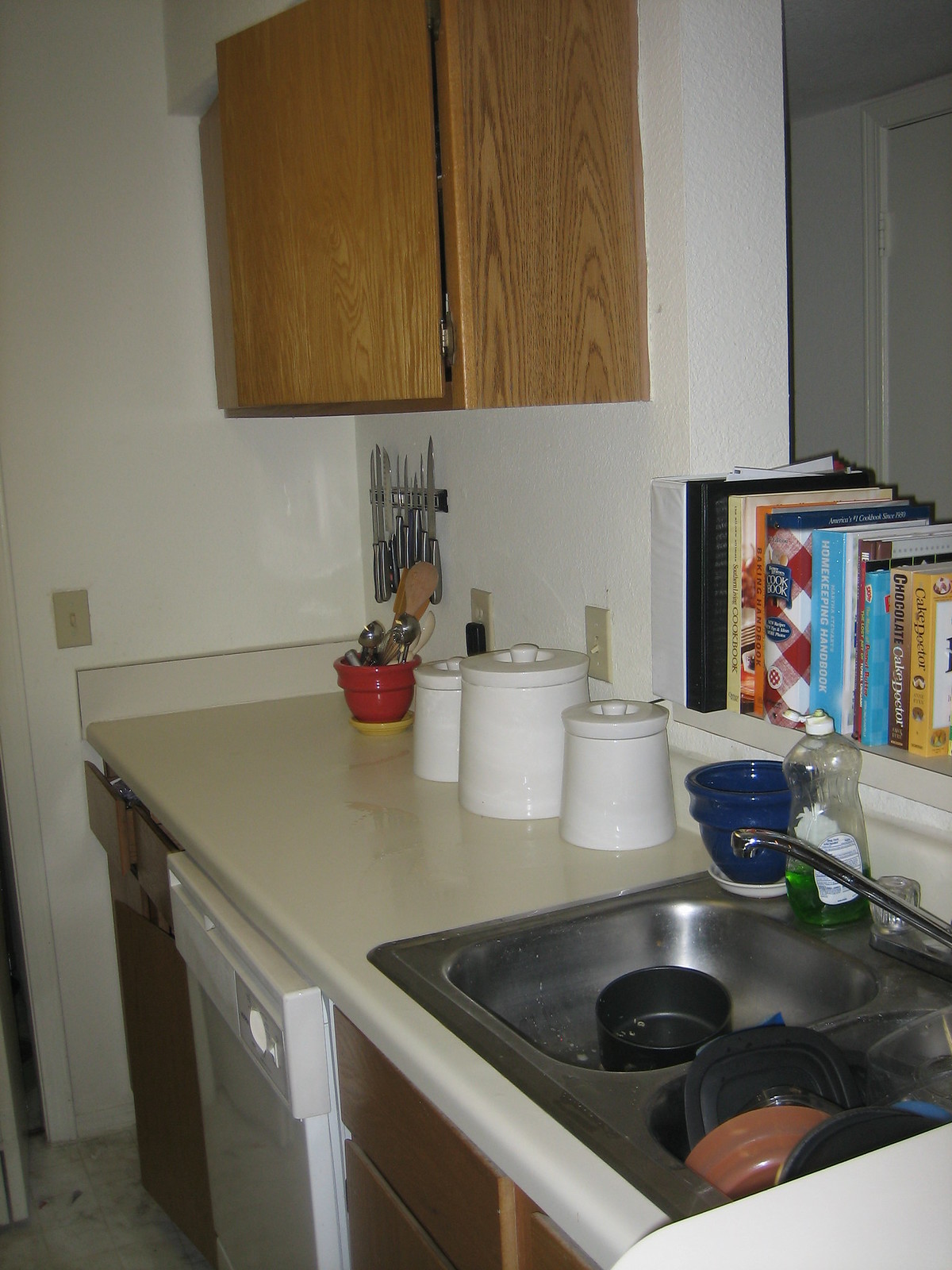The image showcases a cozy, modestly-sized kitchen with a cream-colored laminate countertop. At the center, there's a double stainless steel sink fitted with plastic turn-knob faucets, characteristic of a vintage 1980s style. The right basin of the sink is cluttered with several black, square food storage containers and a brown pot, while the left basin contains a solitary black pot.

On the countertop behind the sink, a large clear plastic bottle of green dish soap, likely Palmolive, stands prominently. Adjacent to it, an empty blue plant holder rests in a white dish. To the left, three circular, white canisters are neatly arranged. On the far right end of the countertop, a red planter pot, nested in a yellow dish, serves a dual purpose by holding various kitchen utensils including a wooden spoon and some smaller stainless steel spoons. Despite the somewhat cluttered appearance, the kitchen exudes a homey and utilitarian charm.